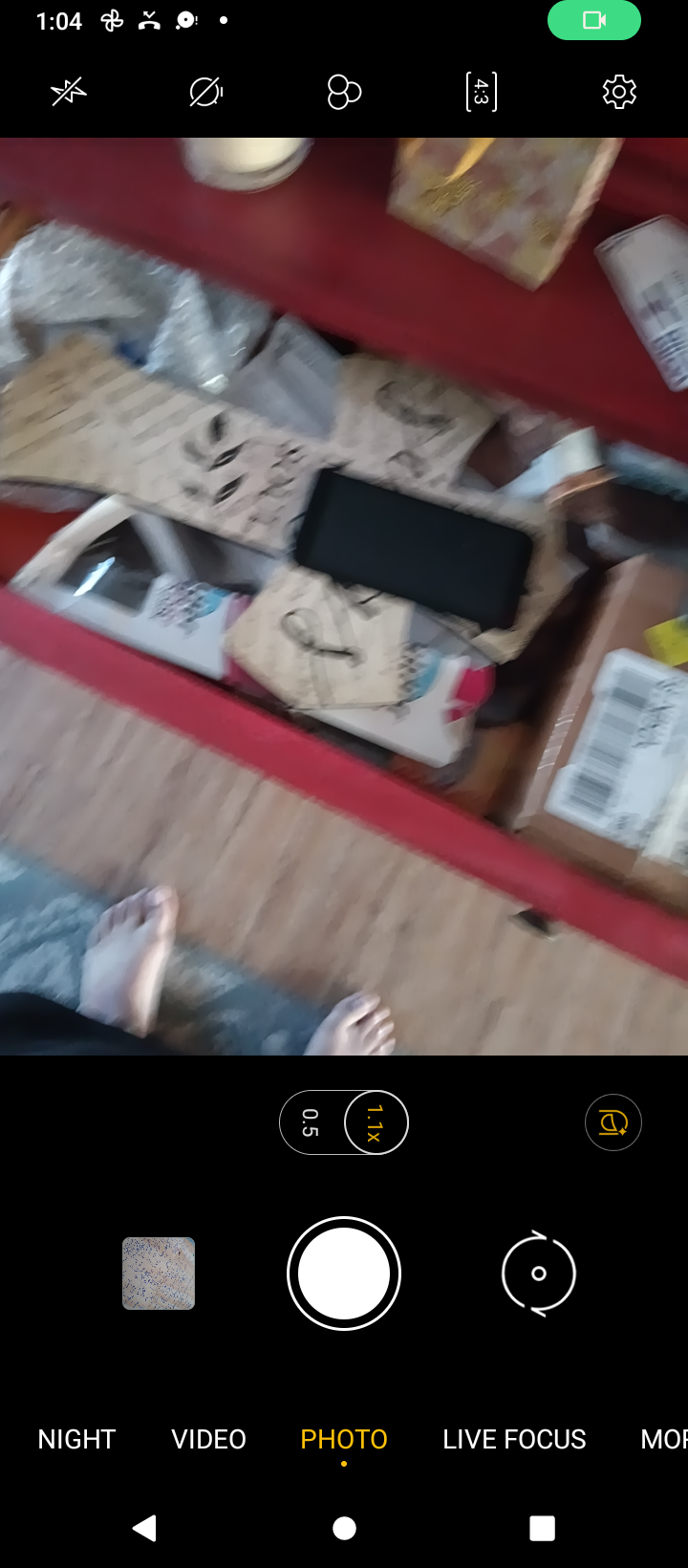The image is a screenshot taken from a phone displaying the camera interface. At the bottom of the screen are the familiar camera function buttons and labels, including "night," "video," "photo," "live focus." At the top, the symbols and time "1:04" are visible, characteristic of the cell phone's status bar. The primary focus of the image is a red, wooden chest with one of its drawers open. On top of this chest rests a round-shaped white object and a square item that appears to be a purse, identifiable by an orange handle extending from it. The contents of the drawer include various items, but due to the blurriness of the image, specifics are difficult to ascertain. Visible is a black rectangular object and a packaged item with its label still attached. The chest's drawer features a visible knob. In the foreground, two feet, oriented towards the chest, stand on a blue rug laid over a light wood floor.